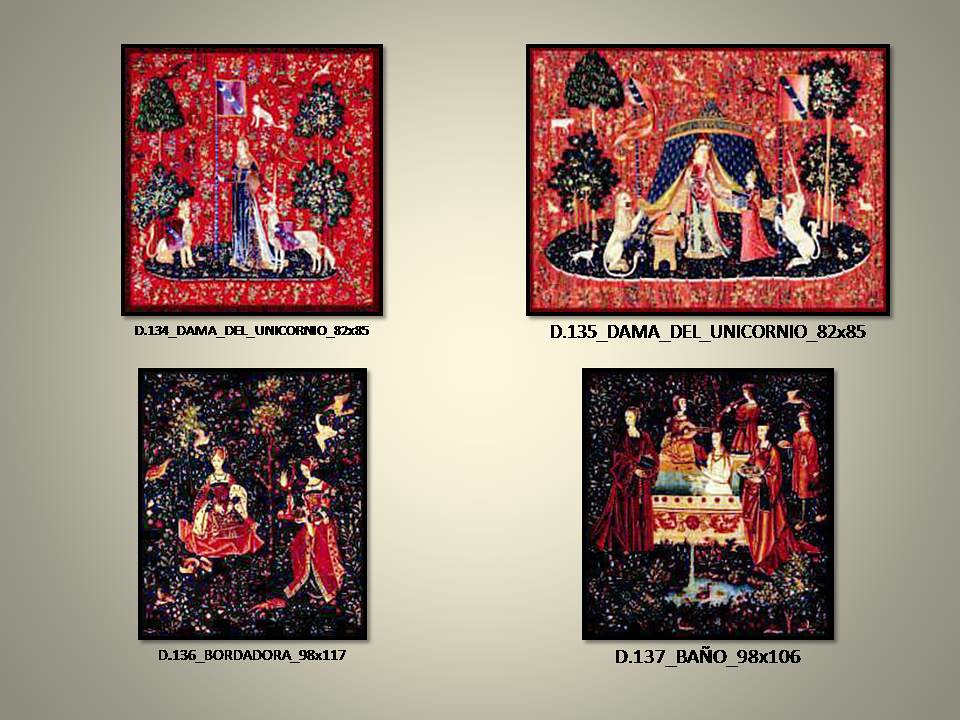This image captures a collection of four distinct, seemingly ancient paintings with a rich medieval and Victorian aesthetic, displayed against a light gray wall. Each painting is defined by a unique yet cohesive color scheme of red and black, embellished with intricate details of flora, fauna, and human figures. 

In the top left painting, set against a vibrant red background with abstract trees, a woman in a flowing, purplish-blue dress stands prominently, holding a red flag adorned with three crescent moon shapes on a black field. Accompanying her are two animals—one that resembles a large dog and another a unicorn—both white and draped in the same insignia as the flag.

To the right, the top painting also showcases a bright red background and features a woman clad in a dress, situated in front of a tent and surrounded by two white unicorns, each marked by the crescent moon flag. 

The bottom left painting, contrasting with a dark black background, presents a scene with two women in red dresses, one of whom is standing, captured amidst a similarly mysterious and medieval setting.

The bottom right painting depicts a group of seven women, all in red dresses, set against another dark black backdrop sprinkled with red and white spots, lending an air of enigma and allure to the scene.

Beneath these intricate artworks is text in Spanish, mentioning titles and dimensions. The top left painting reads "D.134 DAMA DALE UNICORNEO 82X85," the top right "D.135 DAMA DALE UNICORNEO 82X85," the bottom left "D.136 BOR DADORA 98X117," and the bottom right "D.137 BANIO 98X106," each adding a sense of historical and cultural context to this captivating display.